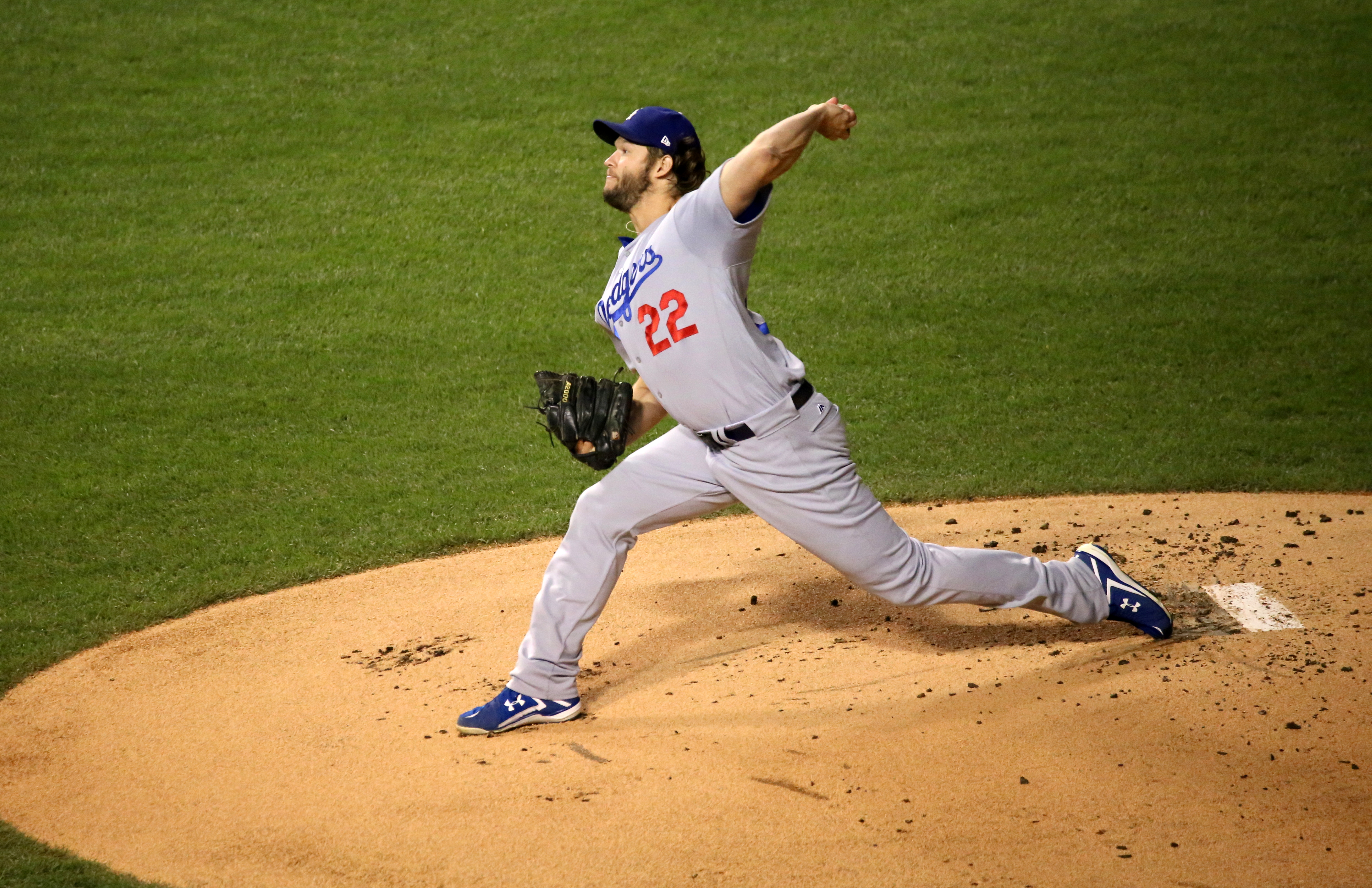This horizontal rectangular photograph captures a baseball pitcher in mid-pitch, centered on the pitcher's mound—a large, circular area of brown dirt. Behind him, the well-manicured infield grass contrasts with the mound. The pitcher, likely a member of the Dodgers, judging by his uniform, wears light gray pants with a black leather belt and a matching light gray jersey adorned with the red number 22 on the front. The jersey also likely features "Dodgers" in cursive blue font across the chest. He is donning blue Under Armour shoes with white bottoms and a blue baseball cap. His left leg is stretched back towards the rubber on the mound, while his right leg lunges forward. His throwing arm, also left, is behind his head, whipping forward with a baseball in hand, and his right hand is encased in a black leather glove. He has medium brown facial hair, adding to his focused expression as he delivers the pitch.